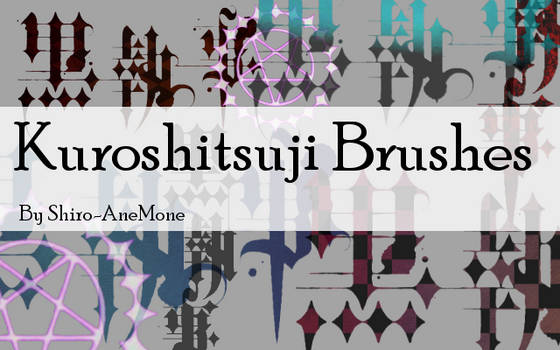This image is a detailed photograph of a logo, resembling the cover of a book or manual. In the center, large black text reads "Kuroshitsuji Brushes," with the 'K' capitalized. Below this, in a smaller font, it states "by Shiro and Monet." The text is placed within a semi-transparent rectangle. 

The background features an array of calligraphy symbols and patterns in a mix of colors—crimson, light pink-purple, and light teal—contrasting elegantly against a light gray, velvet-shaded backdrop. Additionally, there are lines and diamonds woven throughout, with notable pink pentagrams in the bottom left and center of the image, the latter being slightly smaller.